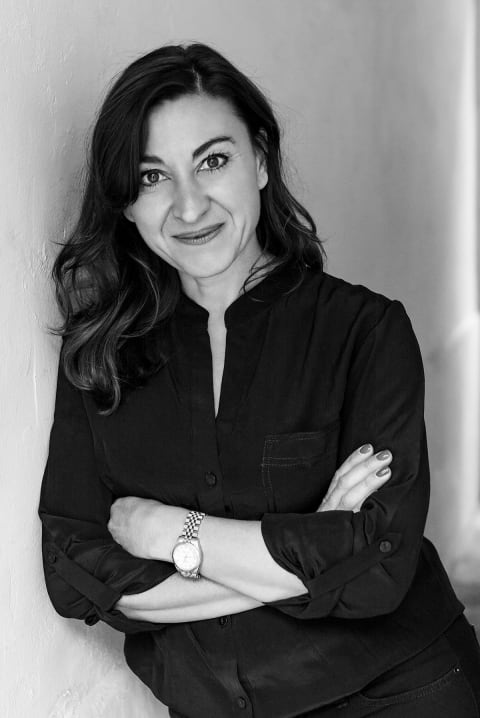The black-and-white photograph captures a woman leaning with her right shoulder against an off-white wall. She is posing for the camera with a semi-smile that suggests she is happy. She has dark hair that falls just below her shoulders, cascading over her right shoulder and tucked behind her left ear. The woman is wearing a black button-up shirt featuring a single pocket on the upper left side and dark jeans. Her arms are crossed, revealing a watch with a white face on her left wrist. Her nails are painted, and although the image is monochromatic, there are subtle details like her mascara and possibly a touch of lipstick, suggesting a professionally taken, portrait-like quality to the photograph.